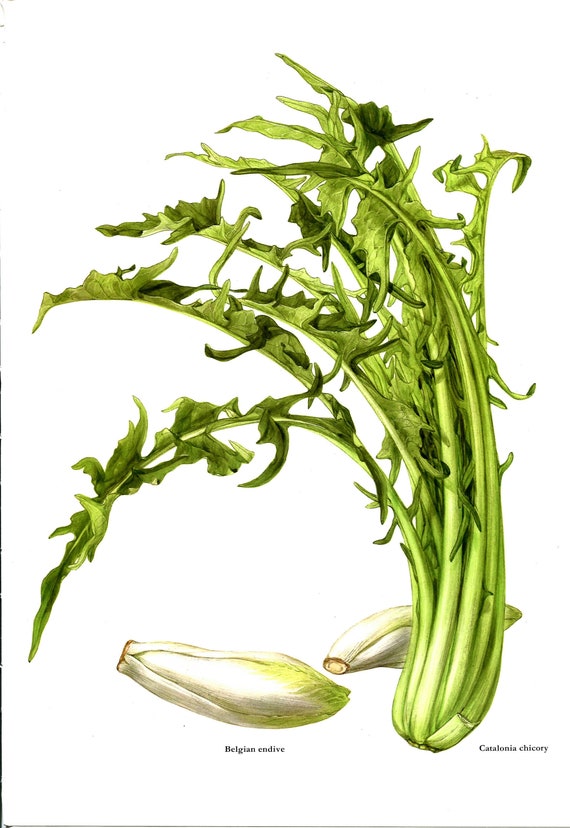This image features a detailed drawing of three distinct vegetables on a white background with some small, barely legible text at the bottom. Two of the vegetables are identified as Belgian endives. These endives, resembling hearts of romaine lettuce, are long, almost rectangular in shape, and have light green tips on their leaves. One of the Belgian endives lies flat with its green leaves fanning out, while the second endive is positioned to the right and partially obscured by the larger vegetable. The larger vegetable dominating the image is a Catalonia chicory. This chicory, reminiscent of celery, has upright, elongated green stalks topped with leafy sections that extend to the very end. The leaves of the Catalonia chicory point leftward, with one leaf drooping over the Belgian endives. The overall composition highlights the Catalonia chicory as the main focus, with the text labeling the identified vegetables as "Belgian Endive" and "Catalonia Chicory."